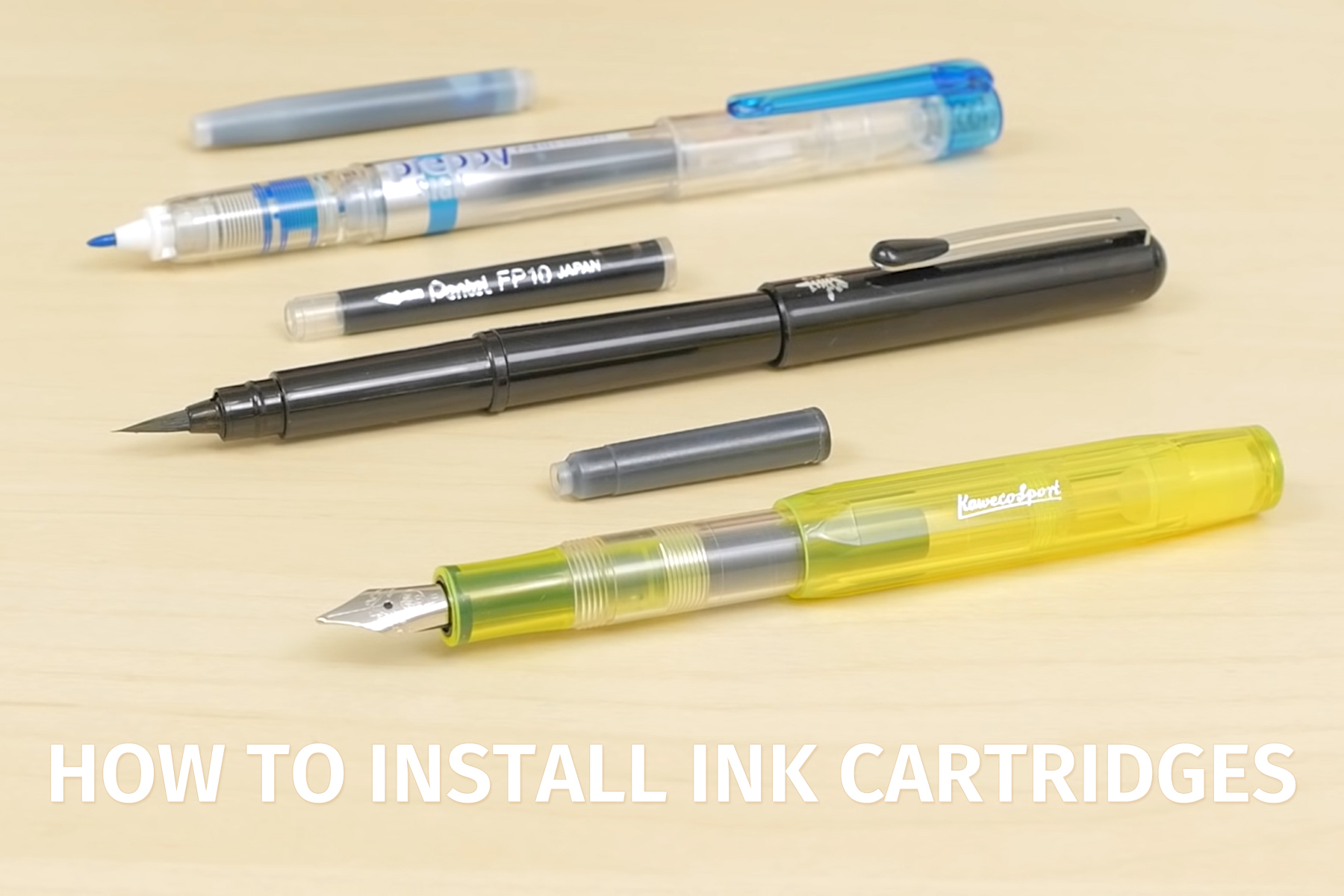The image features three different pens arranged in a vertical line on a light wood-colored or light peach background. Each pen has an ink cartridge positioned next to it, and at the bottom of the image, there is bold white text that reads "How to install ink cartridges."

The topmost pen is primarily translucent with light blue accents on the tip and click mechanism. This pen is likely identifiable by its clear body, allowing visibility of its internal components. Next to it lies a corresponding blue ink cartridge.

The middle pen is entirely black, with a sleek, sharp tip. This pen stands out due to its opaque design and the black ink cartridge that accompanies it. The cartridge has faint, hard-to-read white text, revealing "FP-10" and "Japan," among other obscured details.

The bottom pen is a transparent yellow, reminiscent of a classic highlighter but with a tip akin to traditional ink pens seen in old movies. The yellow pen is paired with a similarly colored ink cartridge that bears white cursive script, possibly reading "Kawako Port," although the stylized cursive makes it challenging to decipher fully.

In summary, the image instructively showcases three distinct pen types—one translucent blue, one solid black, and one transparent yellow—each with their own specific ink cartridges, all set against a light background with a clear instructional label at the bottom.